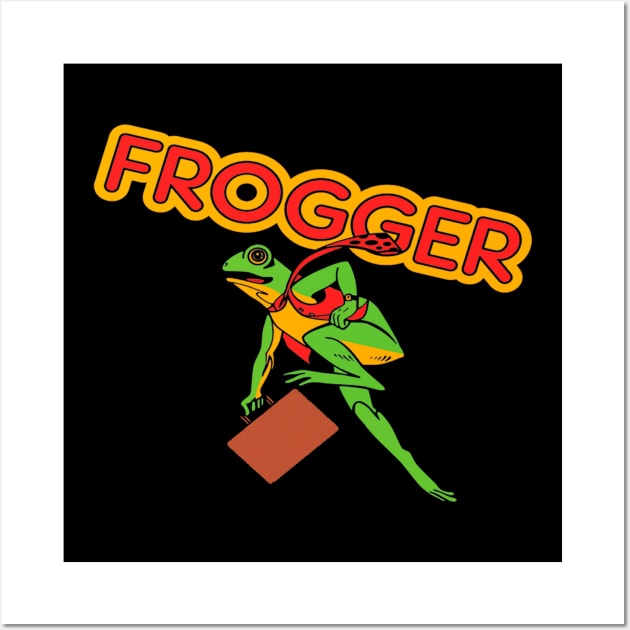This is a vintage game still for the classic video game "Frogger." The image features a black background framed by a thick white border, creating a striking contrast. Prominently displayed at the top in large red bubble letters, the word "Frogger" is outlined with a yellow background. Below the title, a green frog with a yellow belly and bulging black eyes is depicted in a dynamic running stance, suggesting a sense of urgency. His left leg is extended outward while his right leg touches the ground, capturing the motion. The frog wears a red tie with black polka dots, which appears to be billowing behind him as he runs. In his right hand, he clutches a brown briefcase. His slightly parted mouth adds a touch of personality, making the overall composition both lively and engaging.